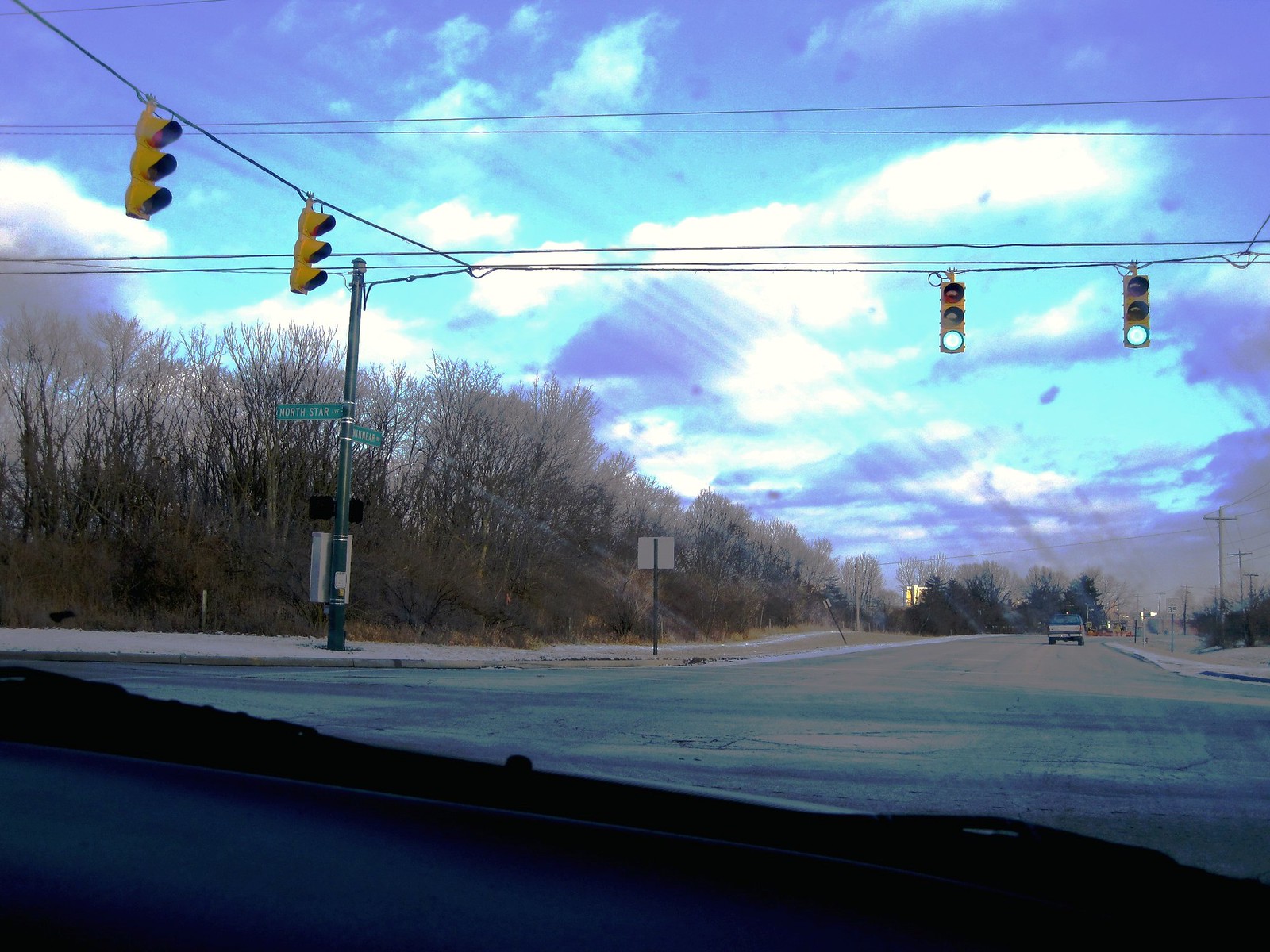The image is a first-person POV taken from inside a car, showing part of the dashboard at the bottom edge, spanning from left to right, and the black windshield wipers lying flat on the windshield. It captures a street scene at a T-intersection, with a mostly empty road ahead. A pickup truck is visible in the distance, approximately 20 to 30 meters away. There are four traffic lights: two on the right side facing towards the viewer and two on the left side facing away. The traffic lights are green. The scene includes a sidewalk on the left with numerous leafless trees in the background atop a small, orange grassy hill. A small rusted pole with green address signs can also be seen. The sky is light blue with a mix of white and dark green clouds, possibly due to the lighting angle. There are no people or animals in the image.